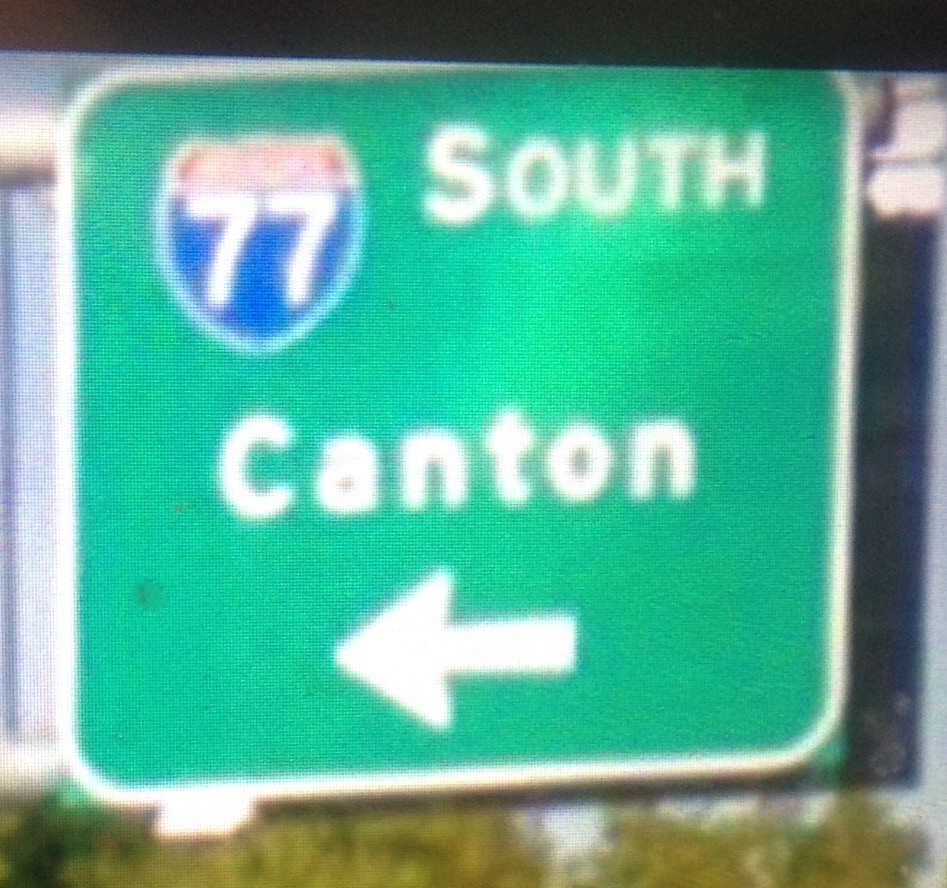This photo captures a close-up of a road sign displayed on a computer screen. The focus is on a large, square road sign with a green background and a thin white border. In the top left corner, the Interstate 77 logo is prominently displayed. To the top right, the word "South" is written in white letters. Dominating the center of the sign, "Canton" is spelled out in large white letters. At the bottom of the sign, an arrow points to the left, indicating direction. There is a noticeable black border at the top of the image, suggesting it is the edge of the computer screen. Horizontal lines run across the entire photo, a result of the image being taken from a computer screen. At the bottom of the image, trees can be faintly seen in the background.